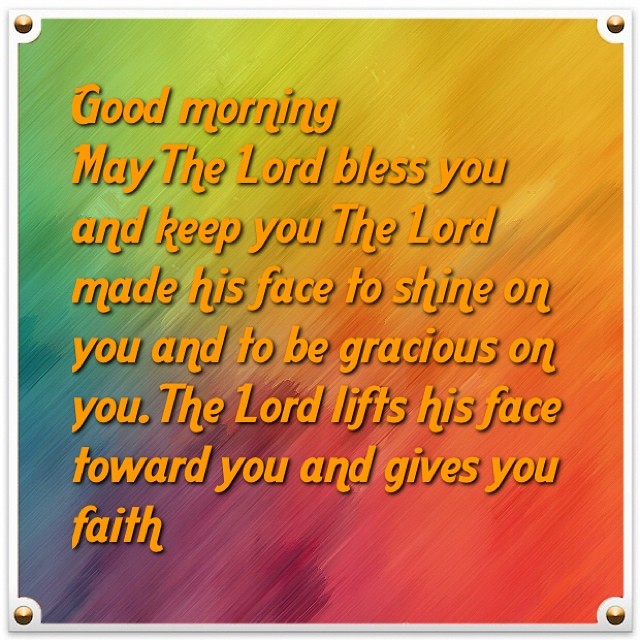This vibrant and inspirational square poster features a religious blessing set against a colorful, gradient background. The background transitions from green in the upper left corner to lighter green and then into shades of orange, purple, and finally red hues in the bottom right corner, resembling a watercolor or colored pencil effect. The text, written in an orange-yellow font, says, "Good morning. May the Lord bless you and keep you. The Lord makes his face to shine on you and be gracious to you. The Lord lifts his face toward you and gives you faith." Each corner of the poster is adorned with graphical representations of gold thumbtacks, adding a touch of whimsy to the design.